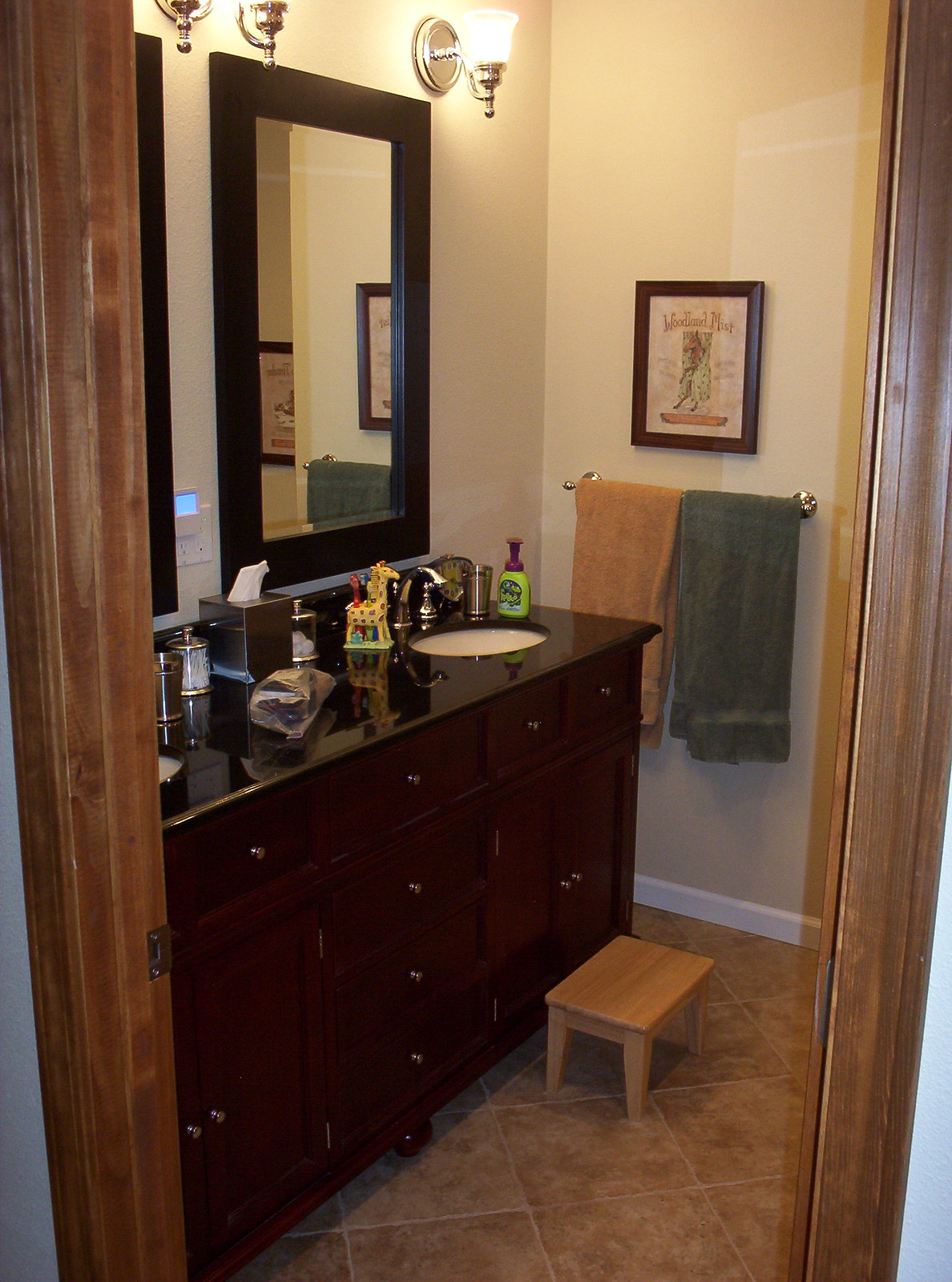This image captures a well-organized and elegantly designed bathroom with the door wide open on the right-hand side. The bathroom features off-white walls complemented by white floorboard molding at the base. The floor is adorned with travertine tiles or a very close look-alike. 

Inside, a dark maroon cabinet with a thick marble countertop takes center stage, holding two white, sunken sinks. Each sink is paired with its own mirror, encased in thick, dark brown frames that coordinate beautifully with the dark wood of the cabinet. The cabinet is functionally designed with two central drawers beneath each sink and four additional drawers down the center, as well as a cabinet under each sink for additional storage.

A small step stool is positioned in front of the sink on the far right, perhaps for a child's use. Atop the counter, practical and decorative elements are present: a giraffe toothbrush holder, a green and purple soap dispenser, and silver hardware faucets. A Kleenex box is flanked by two glass containers, one filled with Q-tips and the other with cotton balls. A mysterious plastic bag rests on the counter, its contents obscured from view.

On the right wall, two towels hang neatly on a towel bar, completing the functional elegance of this inviting bathroom space.